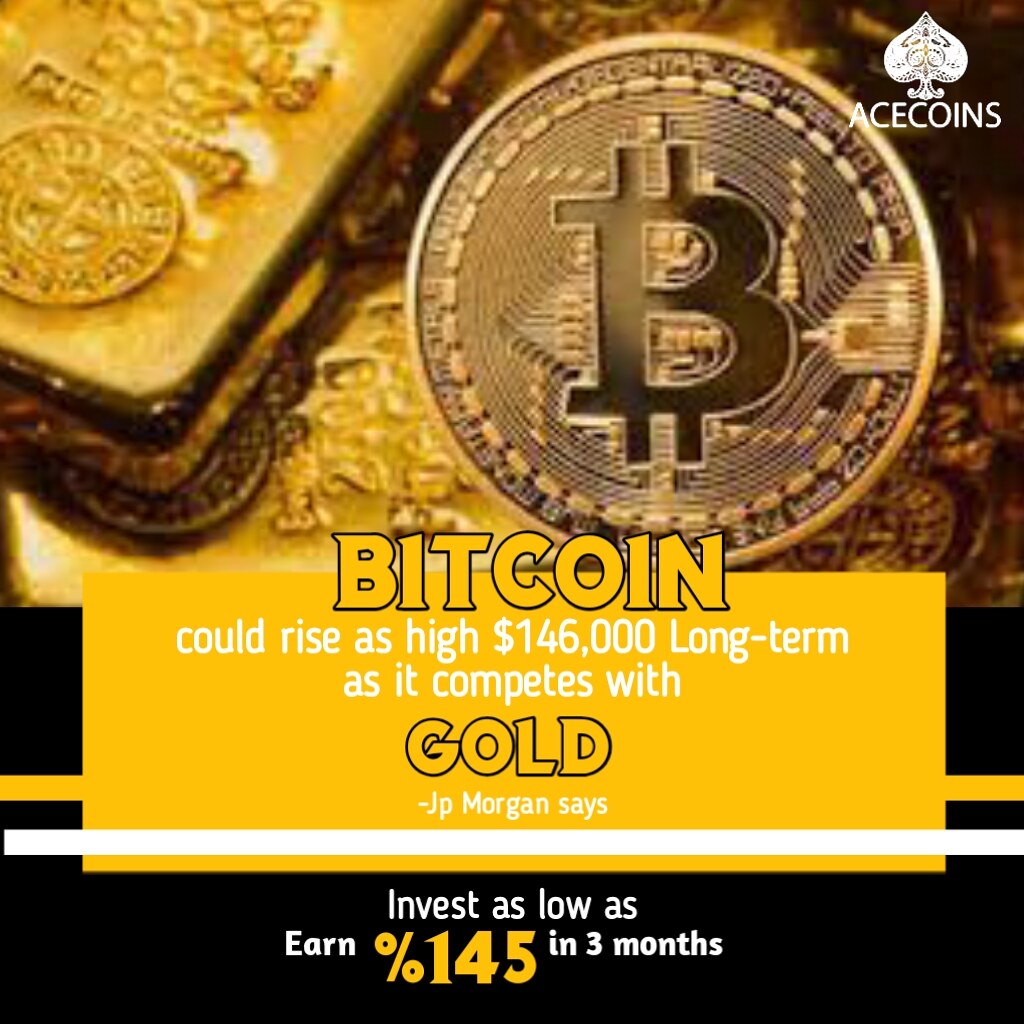This advertisement for Bitcoin, from a company called Ace Coins, prominently features a gold-themed design. Dominating the center-right is a large gold coin bearing the Bitcoin logo ("B"). To the left of this coin are a gold bar and a gold sheet with a design, reinforcing the investment motif. A bold, gold banner stretches across the ad, proclaiming in gold and white text, "Bitcoin could rise as high as $146,000 long term as it competes with gold," attributed to JP Morgan. Below this, in a black banner at the very bottom, it states, "Invest as low as and earn 145% in three months." The entire background consists of stacked gold bars, enhancing the message that Bitcoin may be as valuable as gold. In the top right corner, the company’s logo, Ace Coins, features a spade symbol, indicating their branding. The overall color scheme is gold, yellow, white, and black, creating a striking visual allure to potential investors.